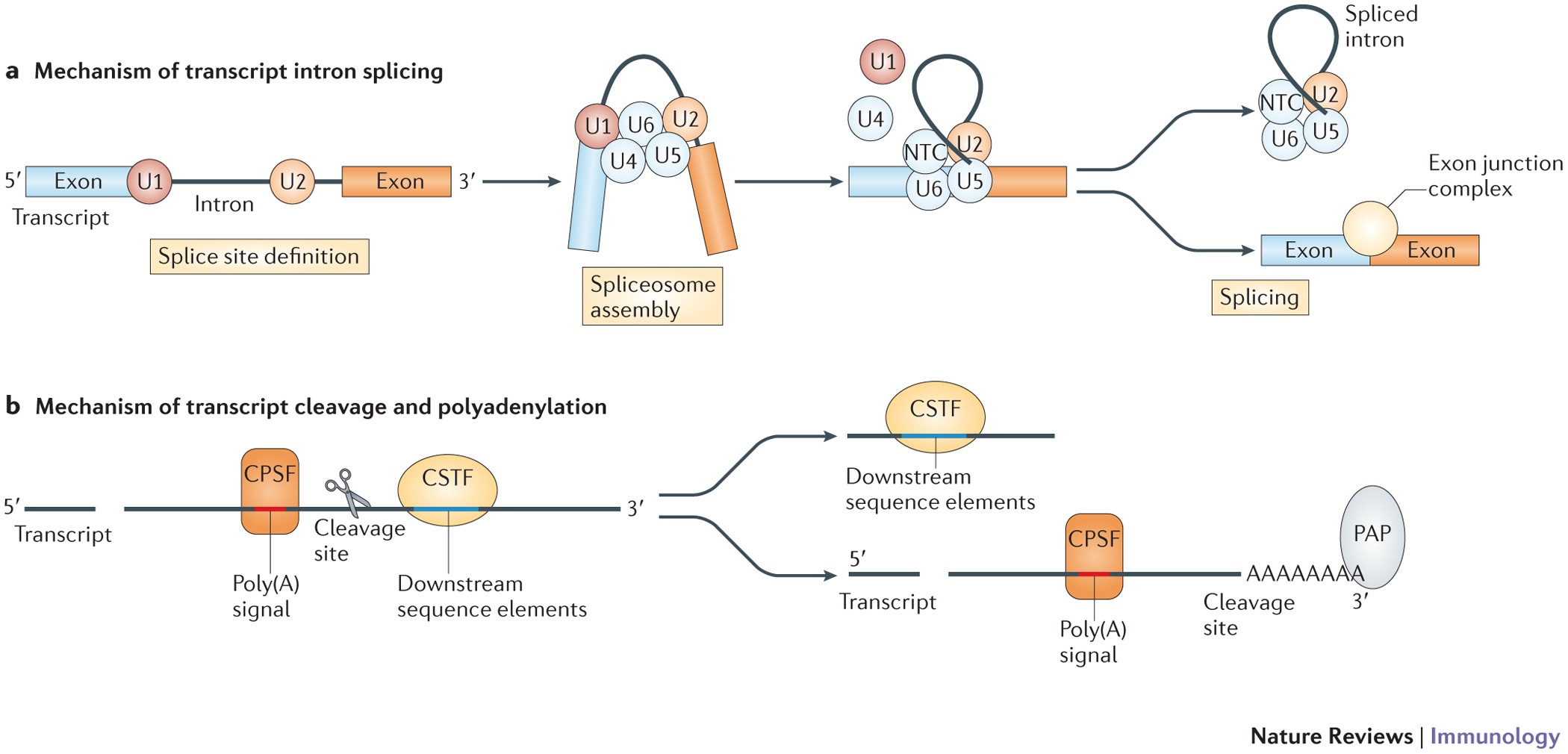The image depicts a detailed scientific chart illustration, divided into two parts labeled A and B. 

Part A, positioned at the top spanning left to right, is titled "Mechanism of Transcription and Splicing." It begins with a label "5'," followed by an Exon depicted as a blue bar marked "U1" in a red circle. Below this, the term "Transcript" is written. The sequence then includes a black line labeled "Intron," followed by another red circle labeled "U2." Continuing right, the sequence features another black bar, an orange box marked "Exon," and beneath all these, a yellow box labeled "Splice Site Definition." The section concludes with another Exon indicated as having a "3'" label.

Part B, situated at the bottom also spanning left to right, is titled "Mechanism of Transcript Cleavage and Polyadenylation." This part includes illustrations of a spliceosome assembly involving components U1, U2, U4, U5, and U6 on a curved structure that ties into progressively more complex knots. The section concludes with a "Transcript Polysignal Cleavage Site" depicted at the bottom right, where scissors illustrate the cleavage point, splitting into two parts. The lower right side is marked with the text "Nature using Immunology."

The image is rendered using colors such as dark orange, pale yellow, light blue, black, white, and various shades of gray, and appears to be styled like a textbook illustration.